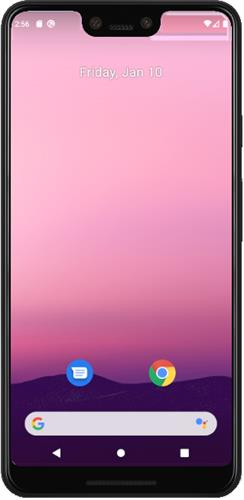This vertically-oriented image captures an Android smartphone encased in a black cover. The screen displays a vibrant pink-to-purple gradient background. At the bottom of the screen, a series of wavy purple mountain-like outlines are drawn. At the top of the screen, white text shows "256" next to two white icons: one resembles a circle with a person inside, and the other is unidentifiable. The typical camera notch is visible in the middle of the top edge.

On the right side of the top bar, the Wi-Fi icon indicates no signal bars, and the battery icon appears fully charged. Centrally placed at the top, in white text, it reads "Friday, Jan 10."

Moving towards the bottom of the screen, there's a blue circle with a white speech bubble icon representing the texting app. To its right is the Google Chrome logo, featuring a red, green, and yellow circle encircling a blue circle rimmed in white. Below this is the Google search bar; at its left is the colorful Google "G" logo, and to its right, a microphone icon, with an empty white space for user input in the center.

At the very bottom of the screen, from left to right, are navigation icons: a triangle (back button), a circle (home button), and a square (recent apps button), all rendered in white.